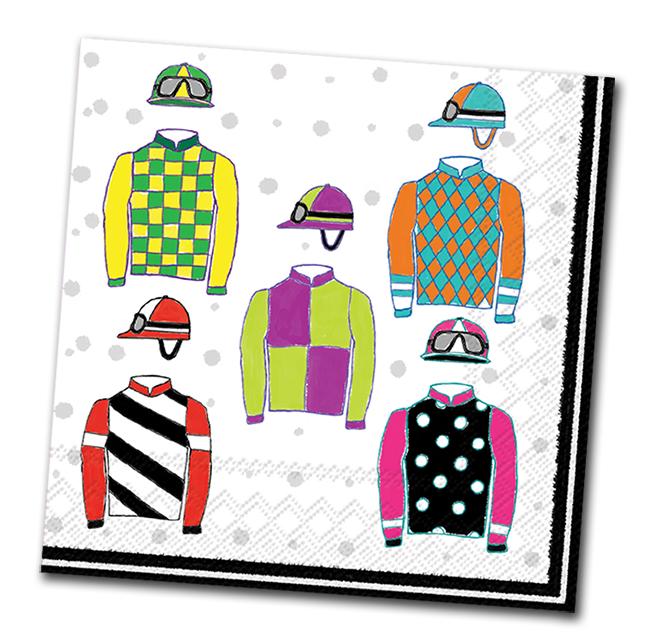The image shows a square, woven fabric object positioned diagonally against a solid white background. The fabric showcases an intricate design featuring five colorful jockey uniforms, each complete with a matching helmet and goggles, reminiscent of classic horse jockey attire. Arranged like the number five on a dice, the vibrant outfits create a striking visual contrast against the backdrop. The upper left displays a checkered pattern in green and yellow, accompanied by a hat in the same colors. To the far right, there is a uniform with a diamond pattern in teal and orange, while the center features rectangular designs in green and purple. The bottom left showcases a red uniform with black and white stripes, and the bottom right is adorned with a pink and black polka-dotted jacket. A subtle detail includes a black border framing the bottom and right sides of the fabric, and small gray dots interspersed throughout the background.